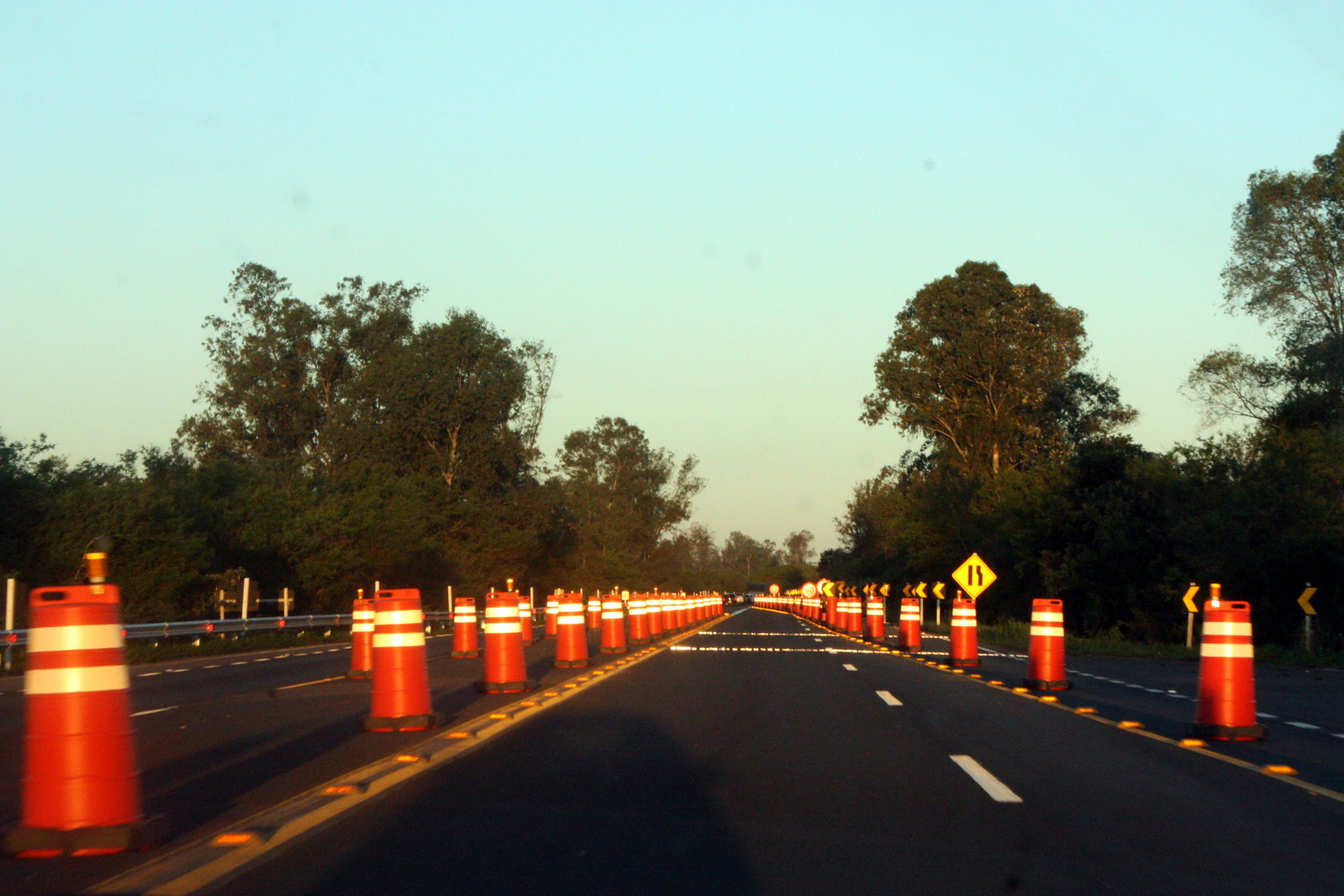This rectangular, landscape-oriented photograph captures a daytime scene at a road construction site. Central to the image is a newly-paved black road, distinctly marked with white lines. Flanking both sides of the road are a series of orange construction barrels, suggesting an active work zone. A prominent yellow merge sign is visible, alerting drivers to upcoming lane changes. In the background, dense clusters of dark green trees frame the roadway, adding a natural border to the construction site. Above, the sky transitions from a light blue hue at the top to an off-white shade near the horizon, hinting at either early morning or late afternoon light.